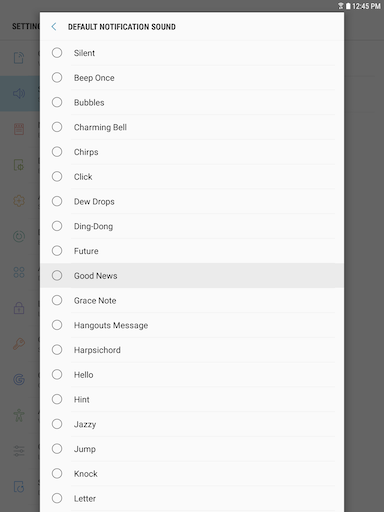The image is a screenshot from a smartphone displaying the settings page for changing the notification sound. In the upper left corner, the time is 12:45 p.m., written in white font. The battery icon is also visible. The rest of the screen is grayed out, indicating the presence of a pop-up box.

The pop-up box, a long vertical rectangle, showcases the section for selecting the default notification sound. At the top, in dark gray bold capital letters, it reads "DEFAULT NOTIFICATION SOUND." Below, there is a list of sound options with small circles next to each choice, allowing users to select their preferred notification sound by tapping on the respective circle.

The visible options, written in gray font and aligned in a column on the left side, include:
- Silent
- Beep Once
- Bubbles
- Charming
- Bell
- Chirps
- Click
- Dew Drops
- Ding Dong
- Future
- Good News
- Grace Note
- Hangouts Message
- Harpsichord
- Hello
- Hint
- Jazzy
- Jump
- Knock
- Letter

There may be additional options not visible in the screenshot.